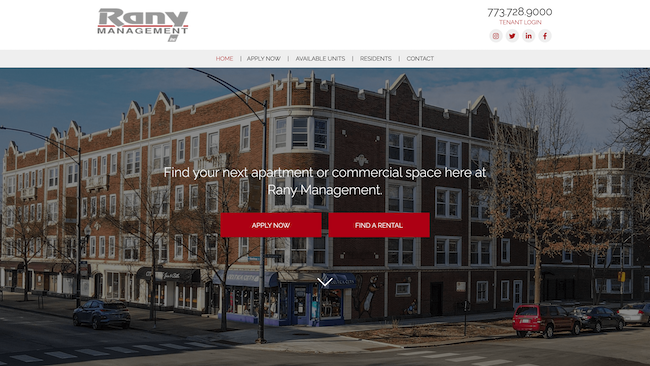This is the homepage for Rany Management (R-A-N-Y), featuring an image of an apartment building with storefronts at the base, situated at a street corner with cars parked along the side. The setting appears to be a sunny fall day, with trees displaying turned leaves that haven't yet fallen. The homepage displays the Rany Management phone number, 773-728-9000, and includes red text for tenant login, along with icons for Facebook, LinkedIn, Twitter, and Instagram. Navigation tabs labeled Home, Apply Now, Available Units, Residents, and Contact are prominently displayed. Overlaid on the image is the tagline, "Find your next apartment or commercial space here at Rany Management." Below this, two red buttons with white text prompt users to "Apply Now" on the left and "Find a Rental" on the right.